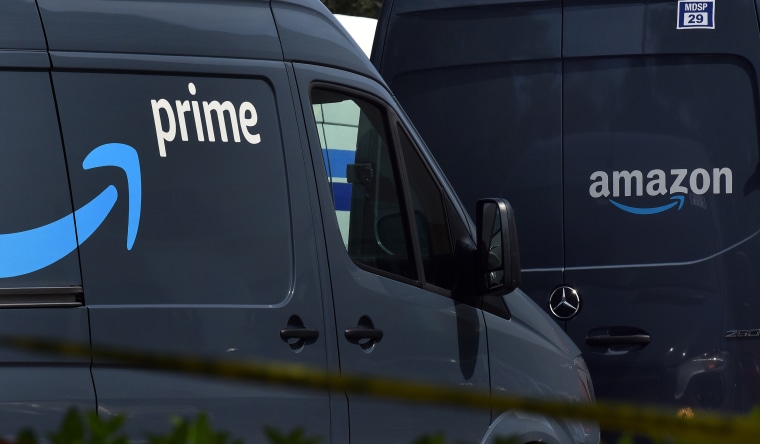The image features two large black delivery vans parked bumper-to-bumper, likely preparing to be loaded with packages. The first van prominently displays the word "Prime" in bold white letters, accompanied by a blue logo resembling a smiley face with an arrow tracing from left to right, symbolizing efficient service. The second van is adorned with the "Amazon" logo, featuring a blue swoosh from the 'A' to the 'Z,' symbolizing the company's comprehensive range of products. Both vans are of the Mercedes-Benz brand, evidenced by the logo on the rear of one of the vans. Additionally, this van bears a blue MDSP sticker with the number '29' in white. The backdoors of the vans are equipped with black handles designed for easy access to the cargo area.